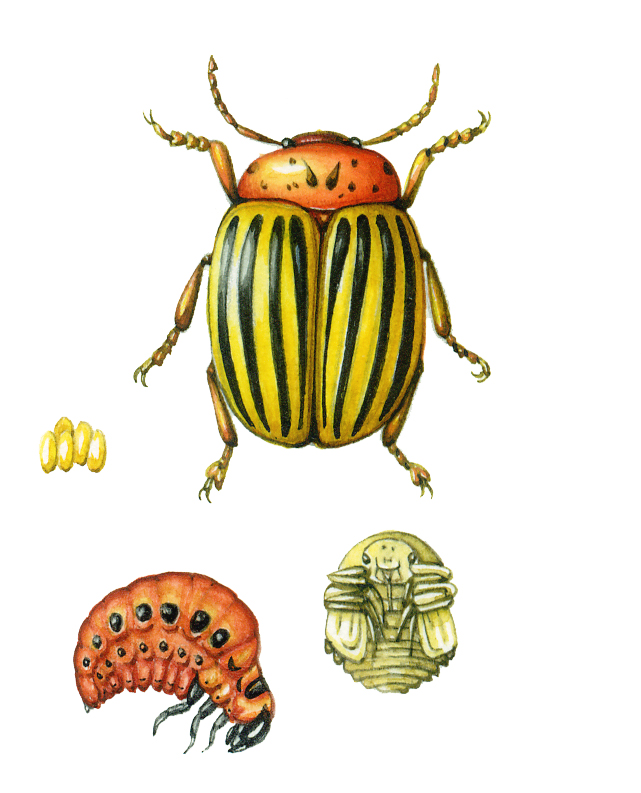The image depicts a detailed artistic rendering, perhaps a digital painting, of three different bugs against a stark white background. At the top of the image is a beetle with distinctive dark orange-colored head and black eyes. Its body features vivid yellow sections with black vertical stripes running from the head to the back. The beetle's legs, which are a dark orangish-brown color, are symmetrically placed with two at the front, two in the middle, and two at the rear on either side. Additionally, it has two antennae of the same dark orange hue extending from its head.

Below the beetle, to the left, is a dark reddish-orange larva, arched upwards. This larva displays horizontal rows of black dots along its sides and has a black head with three black legs.

To the right of the larva lies another creature, depicted in pale yellow shades. This bug has an almost shield-like shape, characterized by a rounded triangular dome. Its surface is adorned with horizontal lines and it features black eyes, suggesting a face. This yellow insect, detailed with tan and white accents, appears to be yet another life stage of the beetle, showcasing the various phases in the beetle's life cycle.